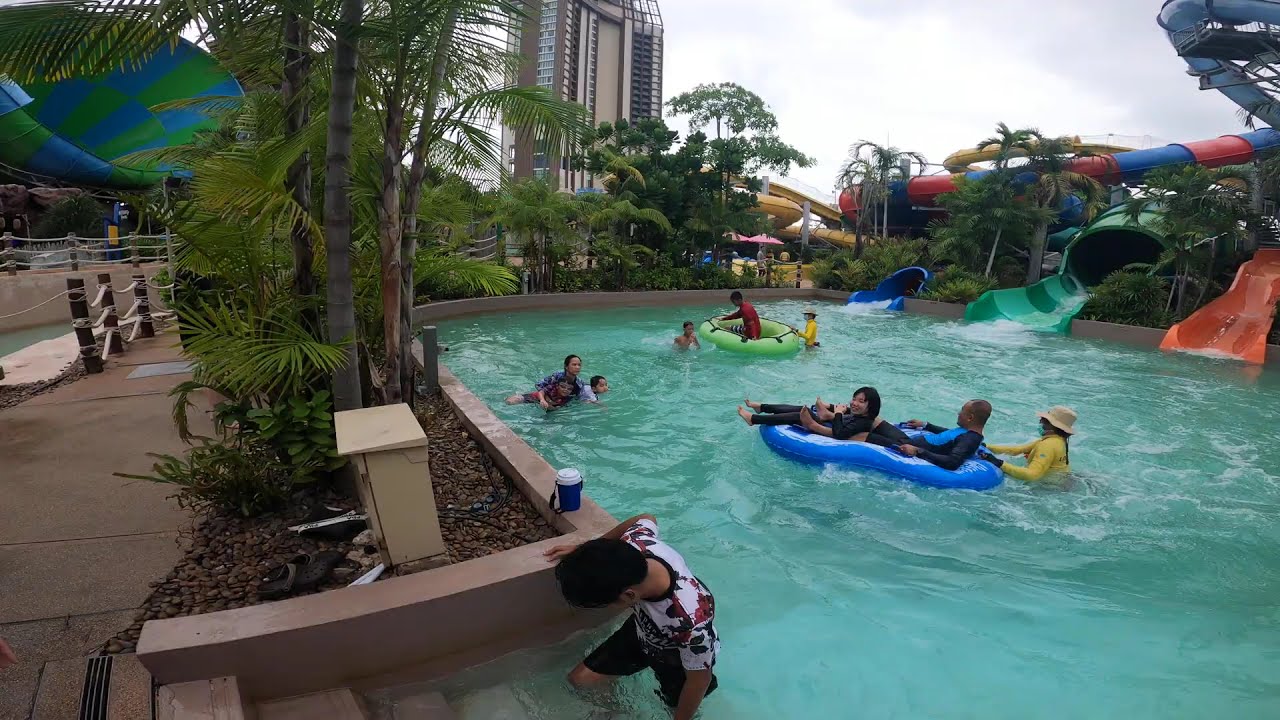The image depicts a lively water park scene centered around a green-watered pool teeming with children and a few adults, floating leisurely on various colored tubes. Dominating the right side of the frame is a vibrant water slide featuring intertwined orange, red, and blue tubes that twist and turn before emptying into the pool. The slides' dynamic structure adds a thrilling element to the atmosphere. To the left, a grand, multi-story hotel towers above, partially obscured by abundant palm trees and other lush shrubbery, enhancing the tropical feel of the setting. In the background, additional slides stretch across different levels, underscoring the expansive nature of the park. Notably, a young boy dressed in a white top with maroon splotches and matching pants is captured walking up the steps towards the hotel. Other park-goers, including a man and a woman on a blue raft and a man with a red shirt on a green raft, are seen enjoying their time in the pool, amidst a backdrop of greenery and further water park attractions.